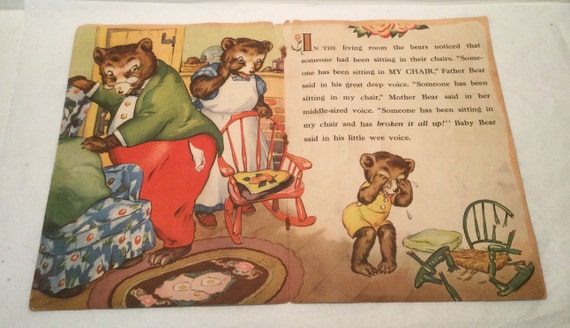This image depicts an illustrated scene from a children's book, likely "The Little Three Bears." The two pages are laid flat and side-by-side, revealing a captivating blend of artwork and text. On the left-hand page, Papa Bear stands prominently in a long gray coat or shirt and red pants, while Mama Bear, dressed in a white apron and blue sleeves, stands slightly behind him with one hand resting on a red rocking chair. In front of them, there's a rug adorned with pink flowers.

On the facing page, Little Baby Bear is portrayed in clear distress, clad in a yellow shirt and shorts, with her hands raised as she cries. Tears stream down her face, drawn in a way that vividly conveys her woe. Before her lies a broken green rocking chair with a wicker seat; its broken back and legs, along with the cushion tossed aside, tell their own story of mishap.

The accompanying text narrates the bears' discovery: "In the living room, the bears noticed that someone had been sitting in their chairs. 'Someone has been sitting in my chair,' Father Bear said in his great deep voice. 'Someone has been sitting in my chair,' Mother Bear said in her middle-sized voice. 'Someone has been sitting in my chair and has broken it all up,' Baby Bear said in his little wee voice."

Papa Bear's chair is described as a comfortable stuffed chair in blue with white flowers and a green pillow, adding to the visual richness. The illustration captures Mother Bear's worried look as she gazes at Baby Bear, whose chair lies broken, emphasizing the overall scene's emotional depth.